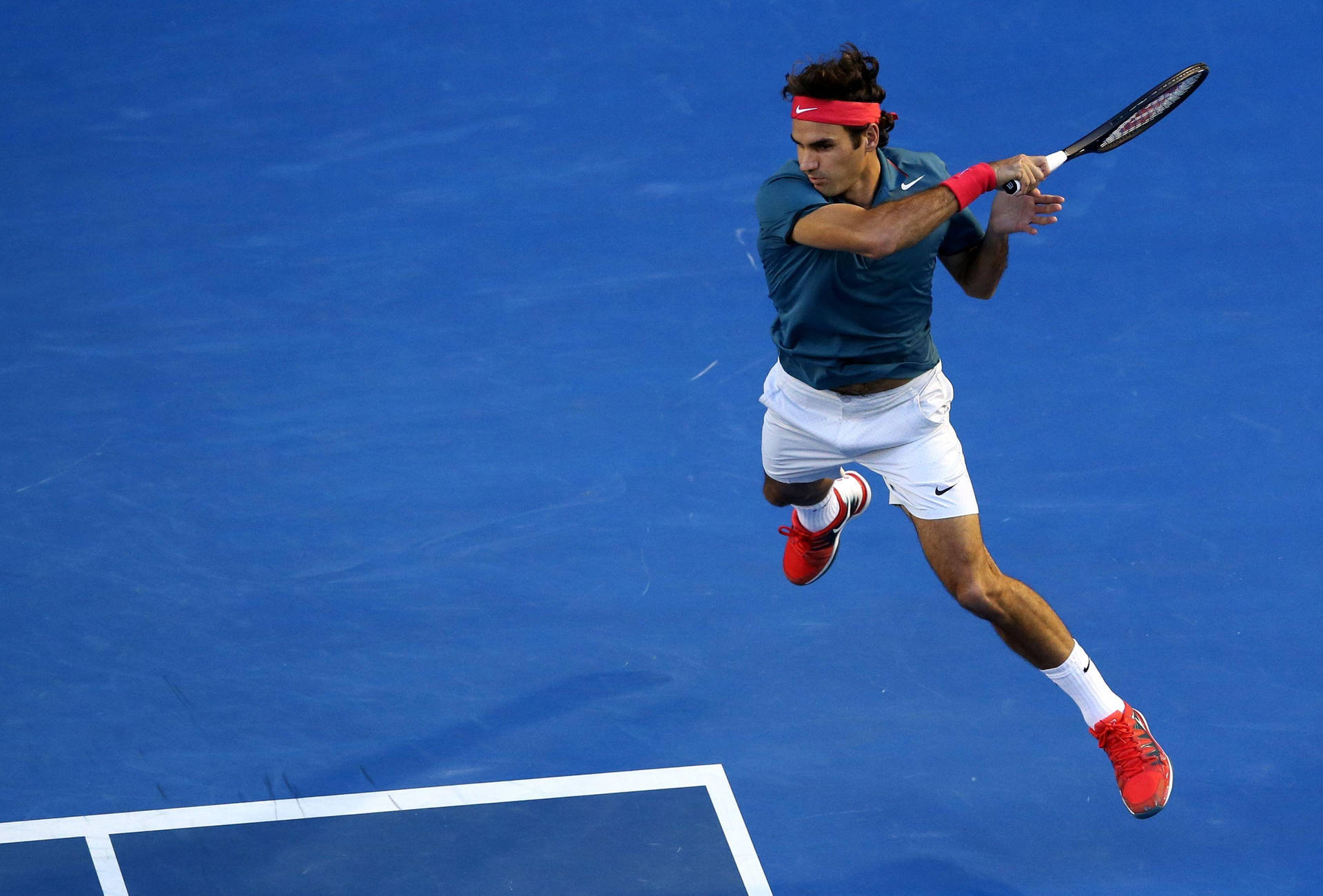In this vivid photograph capturing a moment of intensity on a tennis court, a tan-skinned man with short, dark curly hair is captured mid-air, seemingly after executing a powerful forehand stroke. Although the tennis ball is not visible, the action and focus of the player are palpable. His concentrated expression underscores the seriousness of the game. The man is outfitted in an entirely Nike ensemble: a dark teal short-sleeve shirt, white shorts, and white socks that extend just above his ankles, complemented by red shoes, a red headband featuring the Nike logo, and a matching red wristband. His legs and arms, visibly tan and hairy, add to the dynamic realism of the image. The setting is a strikingly bright blue tennis court, marked by crisp white stripes, which forms the entire backdrop, devoid of other elements or people, thereby focusing all attention on the athlete's impressive leap in the air.